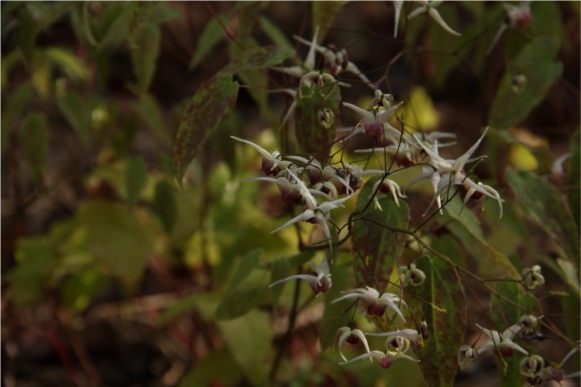The image is a very close-up shot of a dense cluster of peculiar flowers on a plant, either in a garden or a forested area. The main subject, slightly off-center to the right, features numerous white flowers with long, sharp tips resembling a four-pointed star emerging from a purplish-violet bud. Each flower appears either straight or slightly curled, suggesting they may be in various stages of opening. The plant has green leaves arranged like a diagonal plus sign, some as large as a hand, with varying shades of green depending on light exposure. Vines extend across the image to the left and right. The background is blurred and dark, almost black at the top, transitioning to lighter shades of green and brown, with indistinguishable details, emphasizing the flowers as the main focus.